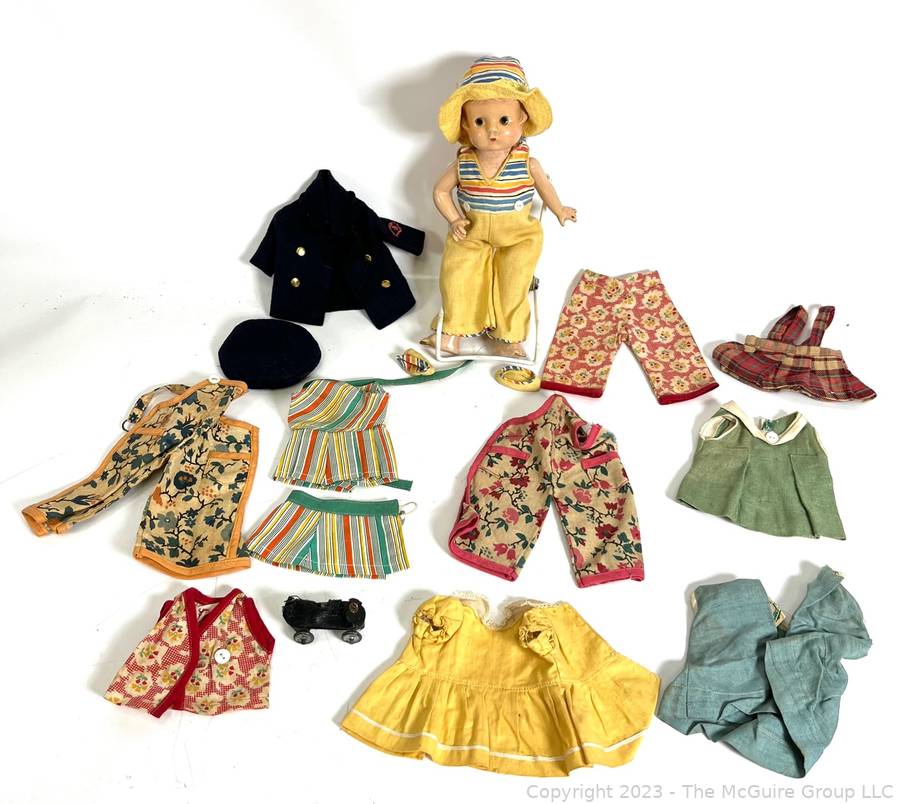The photo displays a white-skinned baby doll situated at the top center against a white background. The doll is adorned in a multi-striped hat featuring a yellow brim, coordinated with a striped outfit in blue, yellow, red, and white for the top half, and yellow pants for the bottom half, complemented by matching slippers. Arranged around the doll are various doll clothes dispersed on the floor, including a black jacket and matching hat, a yellow dress, a green top, red flower-patterned pants, a plaid shirt, blue pants, a green dress with a matching skirt, a colorful striped two-piece set, an orange print two-piece set, and additional items such as a red printed vest, a red cardigan, and a hat. A little doll carriage is also visible among the clothing.